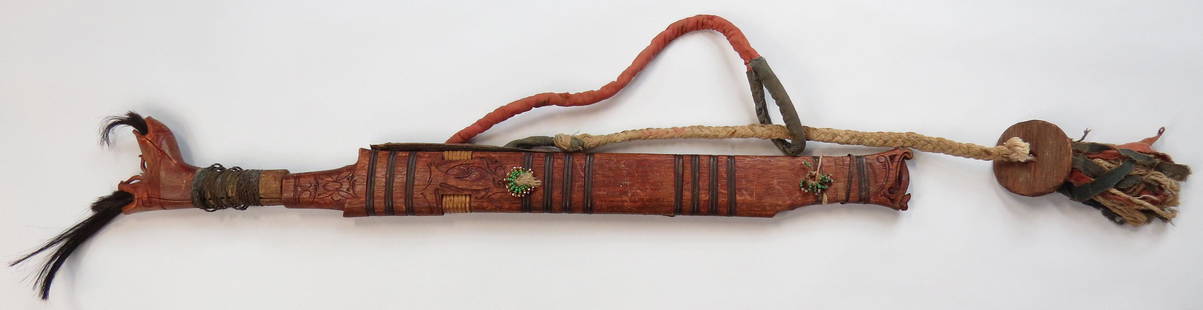The image depicts a primitive, traditional weapon or tool, likely from a Native American or similar ancient culture. The object, made of red wood, features intricate artistry, including green and silver beading and small vertical black lines along its length. It’s long and stick-like, adorned with black feathers or hair at one end. A red rope with a black circle at its end threads through a natural-colored rope, which holds a wooden disc with tassel-like strands. The item, which appears to be in a holster, is set against a plain white background. This historically rich artifact, detailed with various small engravings and additions, evokes the craftsmanship of old, non-modern cultures.